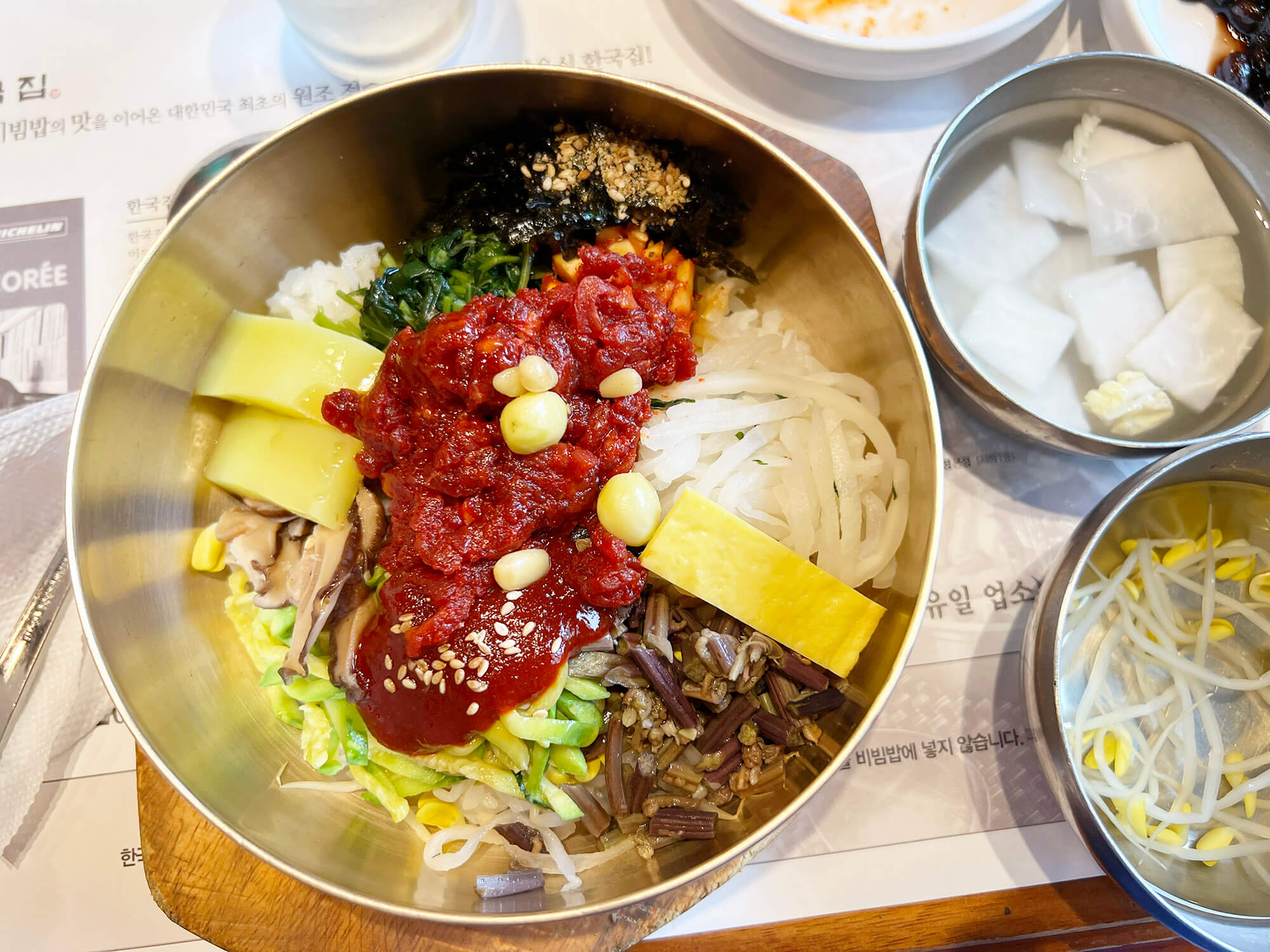In this overhead, realistic photograph, a horizontal arrangement showcases a light wooden table adorned with a white placemat featuring Asian characters. Centered on the placemat are three stainless steel dishes. The main large bowl on the left presents a colorful and diverse meal, featuring white and green noodles, spinach, white rice, and two slices of what appears to be pineapple. This bowl also includes a mix of vegetables such as bean sprouts and cucumbers, and toppings like peanuts or sesame seeds, all accented by a central red sauce. To the top right, the bowl contains white sliced vegetables sprinkled with orange bits. The bottom right bowl holds clear noodles mixed with small yellow pasta pieces. In the very corner, there's a plate with a black substance, possibly garnished with nuts. The scene is subtly accompanied by a barely visible glass of water, and a menu that peeks out in the background, grounding the meal in an authentic Asian dining experience.